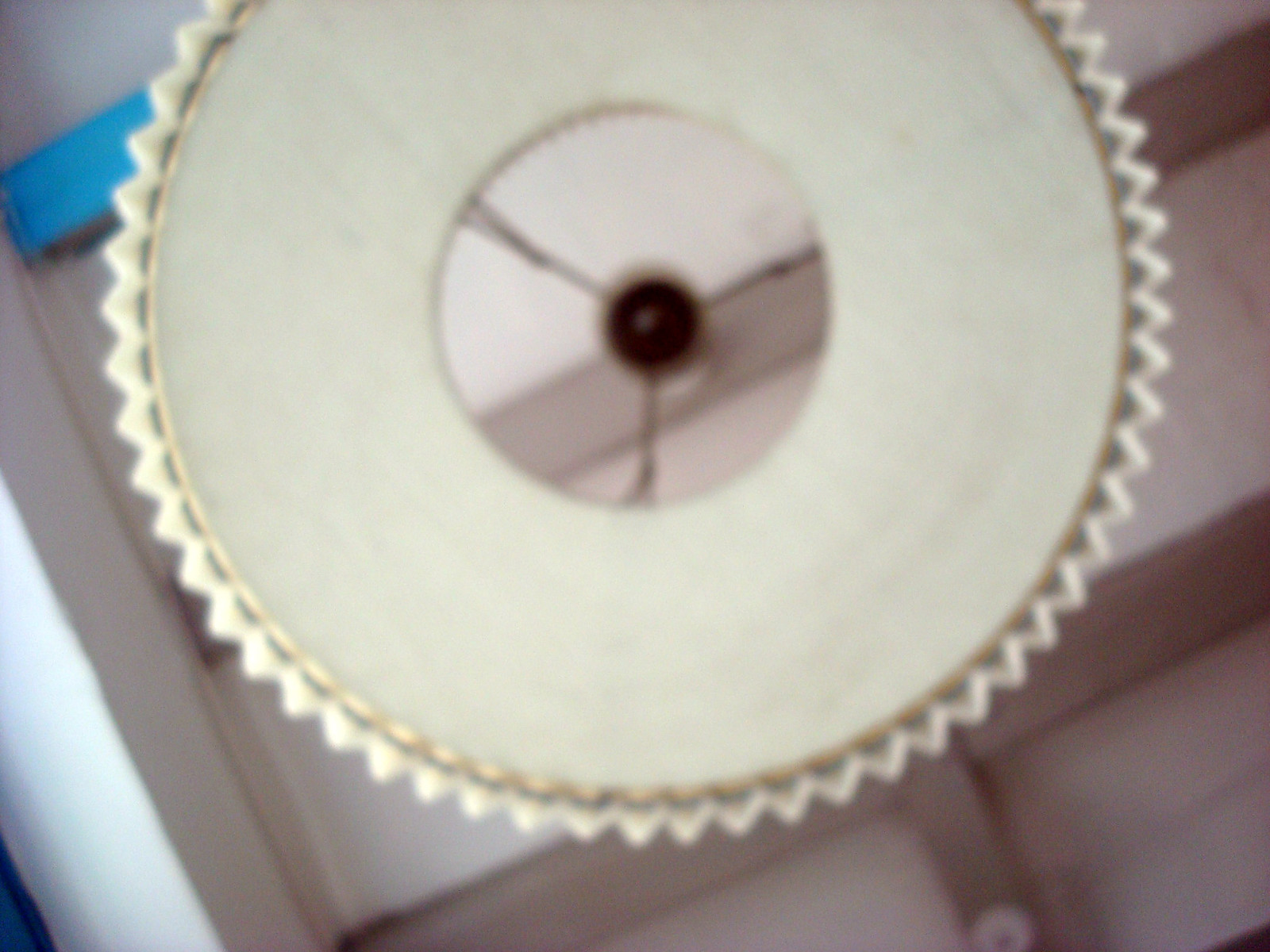The image depicts an indoor scene dominated by a lamp taken from an unusual perspective. From a bird's eye view, you get to see the intricate details of the lamp's socket where the light bulb is screwed in. The photograph focuses on a round, white lampshade adorned with a frilly, lace-like pattern around its bottom edge, which zigzags all the way across. The centerpiece of the lampshade is a gold circular frame featuring a distinct red dot in the middle surrounded by three silver spokes radiating outwards. Though slightly blurry, the image reveals a background with a crisscross pattern that is possibly a ceiling, a table, or even steps, adding an element of spatial ambiguity. Additionally, a blue strip appears on the left-hand side, possibly indicating the edge of the setup or an adjacent object. This composition, intriguing yet puzzling, could easily be part of an art project or a design piece.